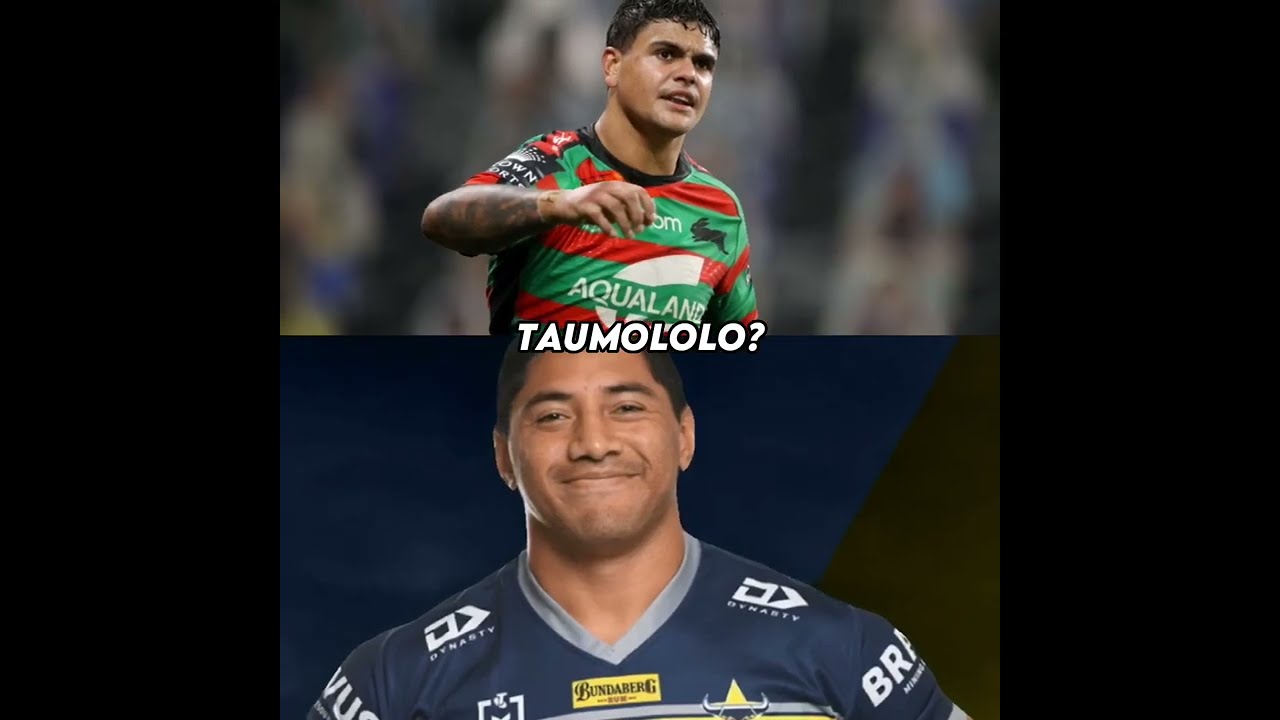The image features a split screen with two distinct photos, each capturing different men who appear to be soccer players. The man in the top image, who has brown skin and short black hair partially covering his forehead, is in action and drenched with sweat. He is wearing a green, red, and black striped jersey with the word "Aqualand" emblazoned in white across the front. The jersey also features an emblem in the upper right corner near his shoulder depicting a black rabbit running left. His arm, which boasts an extensive sleeve tattoo, is raised in front of him, in line with his chest, and his expression suggests he might be celebrating, displaying an open-mouthed smirk. A blurred crowd serves as the backdrop.

Beneath this image is another man with brown skin and black hair, though he is not captured in action. He wears a blue jersey with a gray collar and a distinctive orange-yellow square logo that reads "Bundaberg." His jersey also displays the letters "V-U-S" on the left shoulder and "B-R-A" on the right, with “Dynasty” written over his collarbone. This man poses for the camera with a similar smirk. Between the two photos, the text "Taumalolo?" is prominently displayed.